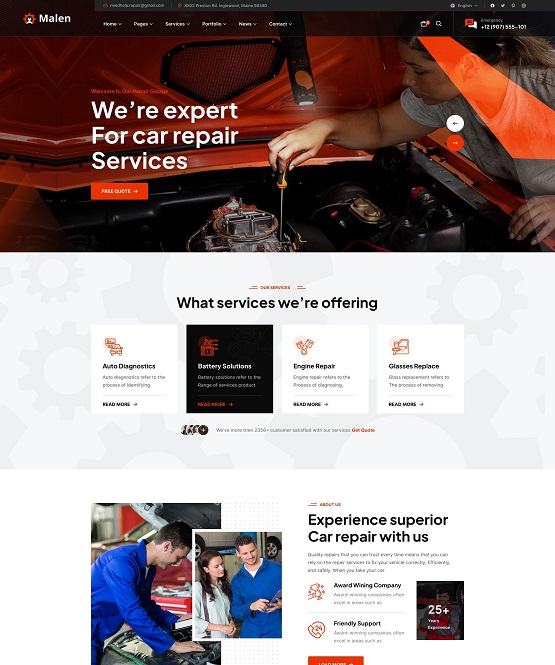This is a detailed screenshot of the website "Malen" which appears to be based in Inglewood, Maine. The homepage features key navigation buttons to various sections including Services, Portfolio, News, and Contact. A search bar is prominently displayed alongside an emergency contact number. The header warmly welcomes visitors with a message: "Welcome to our repair garage. We're experts in car repair services," and features a prominent red button labeled “Free Quote.”

On the homepage, the text “What Services We're Offering” introduces categories such as:

- **Auto Diagnostics:** It describes the process of identifying issues in vehicles, with a “Read More” link for additional information.
- **Battery Solutions:** This highlights services related to battery maintenance and repair, also accompanied by a “Read More” link.
- **Engine Repair:** Another key service area with a “Read More” option.
- **Glass Repair:** Detailing their offerings in fixing car windows and windshields, again with a “Read More” link.

Furthermore, the “About Me” section promotes the company's commitment to superior car repairs, emphasizing quality, efficiency, and safety. It suggests that trusting Malen with your vehicle ensures reliable services every time, accompanied by another “Read More” link.

The website boasts of its credentials as an award-winning company with over 25 years of experience, highlighting qualities such as friendly support. Visuals include images of technicians working on cars and a representative explaining repair costs to a customer, enhancing the narrative of trust and professionalism.